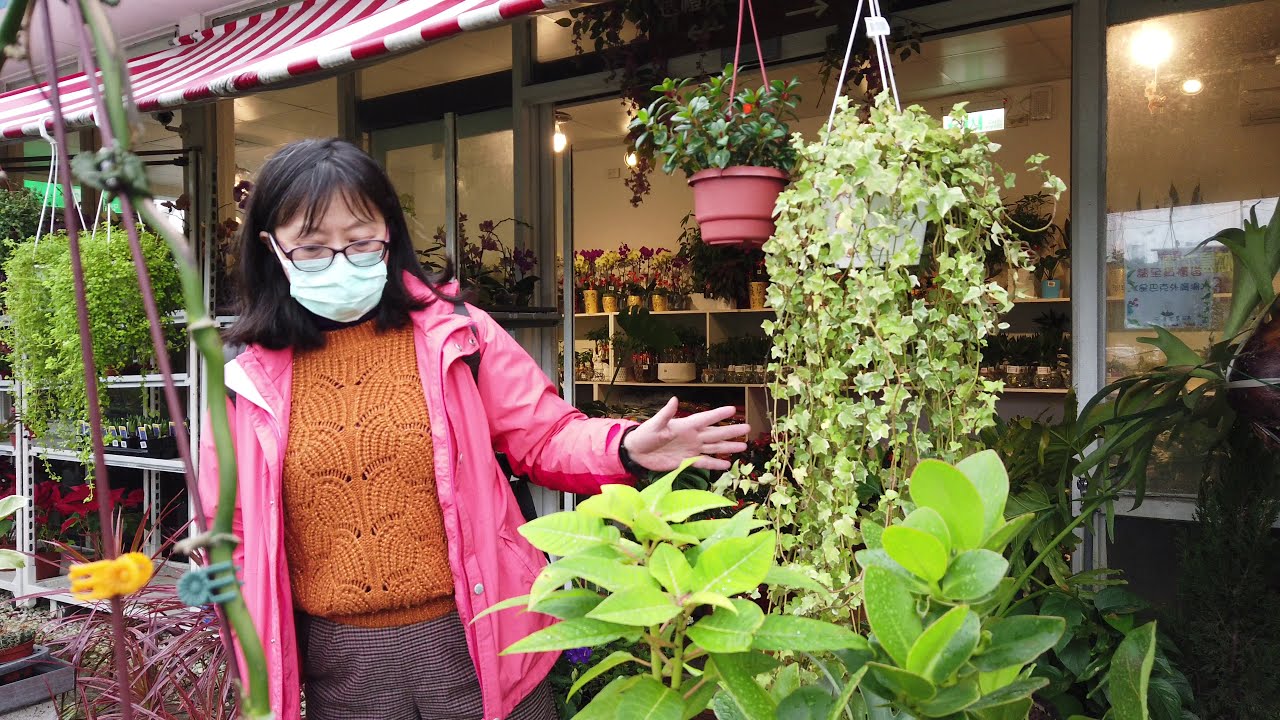The image captures a woman standing outside a plant shop, on the left side of the frame, wearing a blue face mask, black-rimmed glasses, and shoulder-length straight black hair. She is dressed in an orange sweater, a pink jacket, and light brown patterned trousers. The scene is bustling with vibrant greenery; she is gesturing with her left hand extended towards a hanging plant with long, vine-like leaves. She appears to be either explaining or pointing out something specific about the plant, suggesting she might work there.

The woman is surrounded by an array of plants. Directly in front of her, towards the bottom of the frame, there is a plant with medium-sized bright green leaves. In the background, shelves display various potted plants and flowers, while a red and white striped awning frames the shop’s exterior above her. On the right side of the image, part of the shop’s interior is visible through a window, showcasing more shelves lined with pots in different colors. A sign with text in an Asian language is also noticeable in blue and red text. This detailed setting, combined with the woman’s attentive gesture, strongly conveys the lively and organized atmosphere of the plant shop during the COVID era.